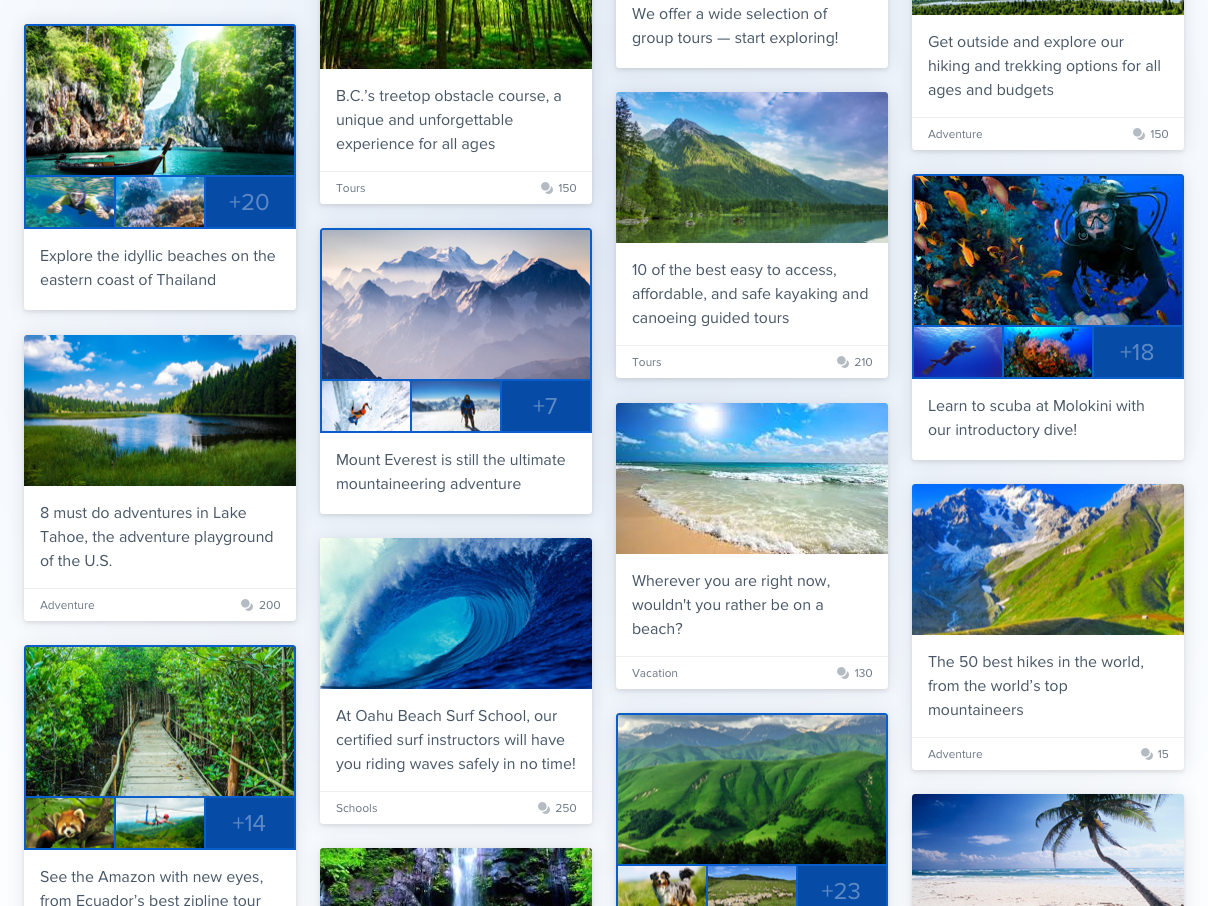This image boasts a light blue background filled with numerous small boxes, each radiating a beach-themed adventure. Here’s a detailed breakdown of the captivating content within each box:

1. **Explore Thailand's Eastern Coast**: This box highlights the idyllic beaches with a serene invitation.
2. **Eight Must-Do Adventures in Lake Tahoe**: Known as the adventure playground of the U.S., this box promises action-packed experiences, accompanied by the number "200."
3. **Amazon Exploration from Ecuador**: Encourages viewers to see the Amazon with fresh eyes, ranked as the fourth best declined tour.
4. **BC’s Treetops Obstacle Course**: Promotes a unique and unforgettable experience for all ages, labeled with "tours" and the insignia "150."
5. **Mount Everest Experience**: Declares Everest as the ultimate mountaineering adventure, showcasing snow-capped mountains.
6. **Oahu Beach Surf School**: Highlights a huge wave and assures that certified instructors will have you riding safely, with a tiny bird icon and the number "250."
7. **Waterfall Image**: An enchanting yet partially cut-off image of a waterfall.
8. **Affordable Kayaking and Canoeing Tours**: Lists 10 of the best easy-to-access, affordable, and safe guided tours, marked with "tours" and the number "210."
9. **Beautiful Beach**: A simple yet profound statement, "Wherever you are right now, wouldn't you rather be on a beach?" with a vacation tag and a numbered circle.
10. **Mountain Image**: Partial image of a striking mountain, tagged with "plus 23" in a blue box.
11. **Outdoor Adventures**: Encourages exploring various hiking and raking options suitable for all ages and budgets, with tags like adventure and a dot.
12. **Scuba Diving at Molokai**: Offers an introductory dive to learn scuba, signifying an underwater adventure.
13. **Top 50 Hikes**: Features the world's top 50 hikes from esteemed mountaineers, with "adventure" and little dots.
14. **Beach Image**: A partially visible image of another enticing beach.

This collage of small boxes collectively promotes an array of adventure-filled destinations and activities, enticing viewers to discover new experiences, from serene beaches and thrilling mountain hikes to exhilarating water sports and immersive treetop courses.